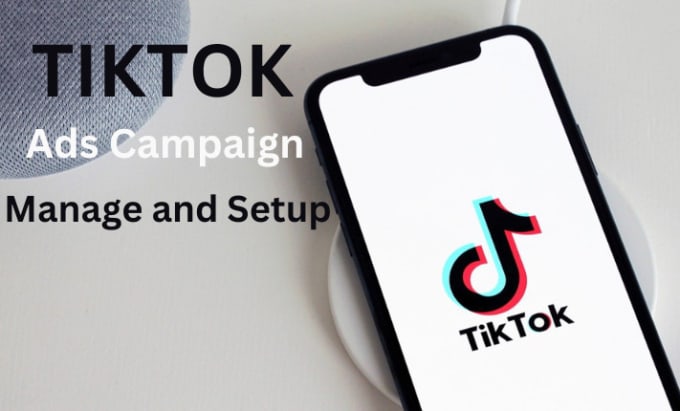Detailed Caption: "The image showcases a TikTok Ads Campaign management setup. At the center, a black-outlined smartphone is prominently featured, encased within a sleek white circular background that includes a black cord. On the phone's white screen, the TikTok logo is distinctly displayed with a black symbol accompanied by a blue accent on the left and a red accent on the right. Below the symbol, 'TikTok' is written in bold black letters. Above the phone, the words 'Ads Campaign' appear in a bold white font, contrasting sharply against the surrounding black font of the other text."